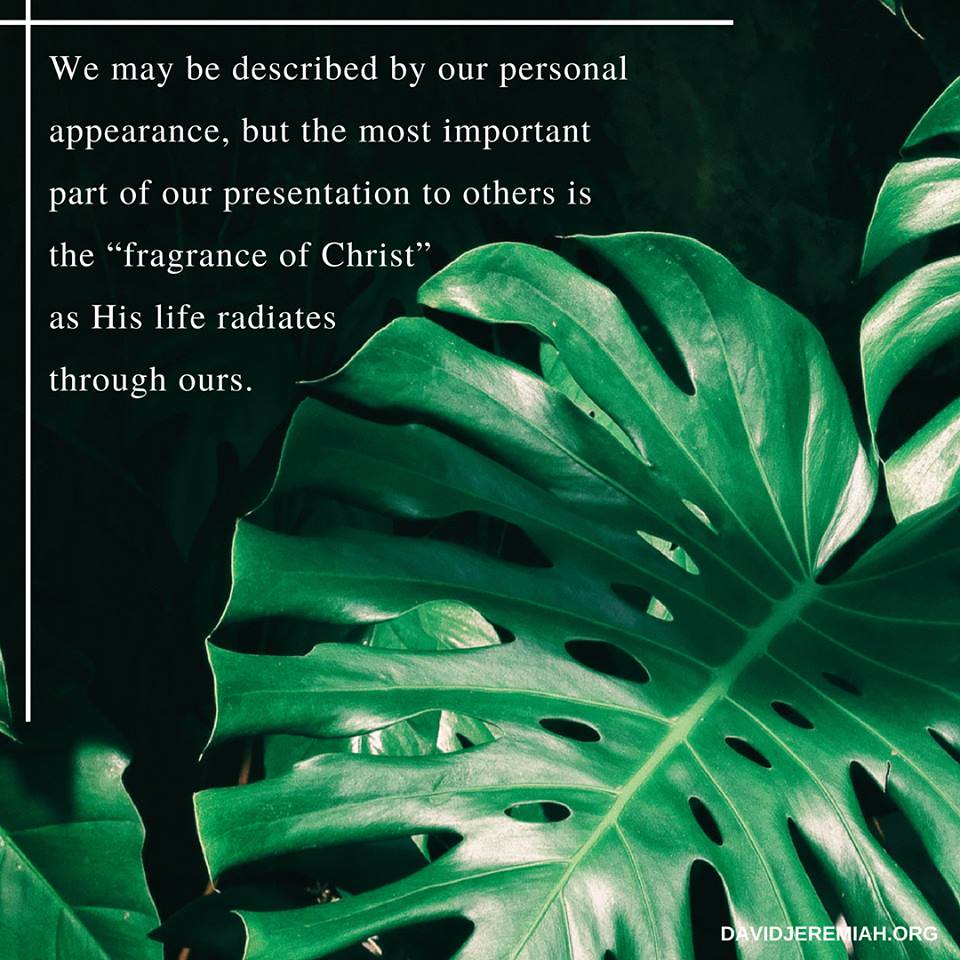The image appears to be a digitally created poster featuring a dark background dominated by a vibrant, detailed close-up of a large green leaf with holes, possibly from a tropical or indoor plant, that spans from the bottom right towards the center. The lower right corner includes the text "davidjeremiah.org" in white. In the upper left corner, overlaid on the black background, is a quote: "We may be described by our personal appearance, but the most important part of our presentation to others is the fragrance of Christ as his life radiates through ours." This text is designed with some decorative white lines, enhancing its visual appeal. The poster, rich in shades of black, white, green, gray, and hints of yellow, appears to be a religious-themed, motivational message intended for social media sharing.